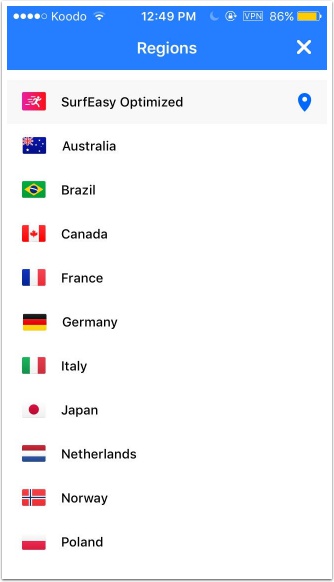This screenshot captures a cell phone interface displaying a regions page. In the upper left corner of the screen, there is cell phone reception represented by four dots, next to the carrier name "Koodo." Adjacent to it, the Wi-Fi icon shows three bars of signal strength. 

At the top center of the screen is the title indicating that this is the "Regions" page. Immediately below, a vertically arranged list of countries is presented. 

The list begins with "Surf Easy Optimized," which features a red icon of a person running to the right. Following are various country names, each accompanied by their respective national flags: Australia, Brazil, Canada, France, Germany, Italy, Japan, the Netherlands, Norway, and Poland.

The time displayed on the device is 12:49 PM.